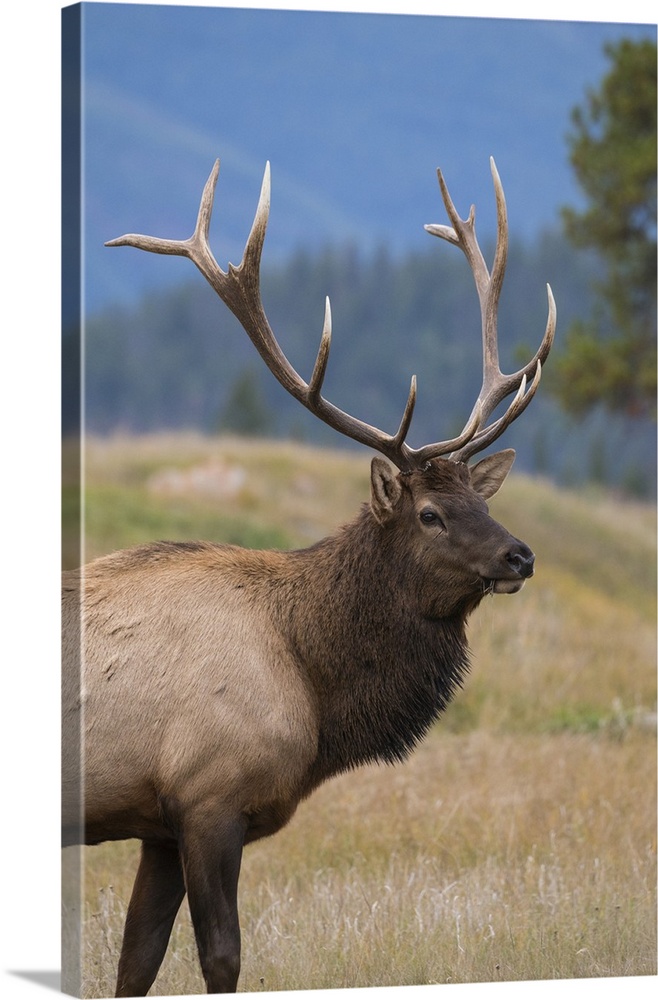"This detailed portrait captures a young male elk with a robust, healthy pair of antlers, emerging gracefully from the left side of a canvas that is in portrait orientation, making it taller than it is wide. The elk's dark brown head and neck transition seamlessly into a tan body, contrasting with its dark brown legs. Standing alert in a field of tall brown grasses with hints of green, indicative of early spring or fall, the elk gazes intently off to the right. In the misty background, which adds a sense of depth and mystery, pine trees and rolling hills blend into the murky distance, partially obscured by the mist that veils the landscape. This exquisite photograph, superimposed onto a wooden-like picture frame for a 3D effect, captures not only the majestic beauty of the elk but also the serene wilderness it inhabits, with towering mountains just barely visible through the mist."